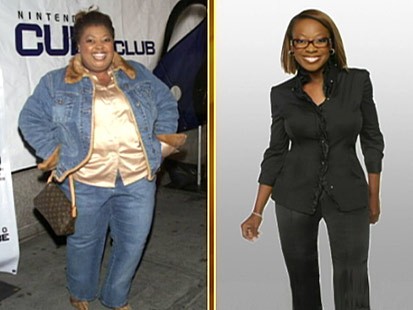This image features a composite of two photographs side by side, each capturing a young Black woman in different settings. On the left, a heavier set woman stands on a carpeted surface, dressed in a blue denim jacket, denim jeans, and a light pinkish shirt, holding a dark purse to her side. Behind her is a white backdrop with partially visible text that includes the words "Nintendo" and "club." On the right, another woman, who is wearing a dark suit jacket and pants, smiles directly at the camera. Both women are the central focus of their respective photos, which appear to depict professional or event settings. The overall color palette of the image includes tones of white, black, brown, blue, tan, and gray.